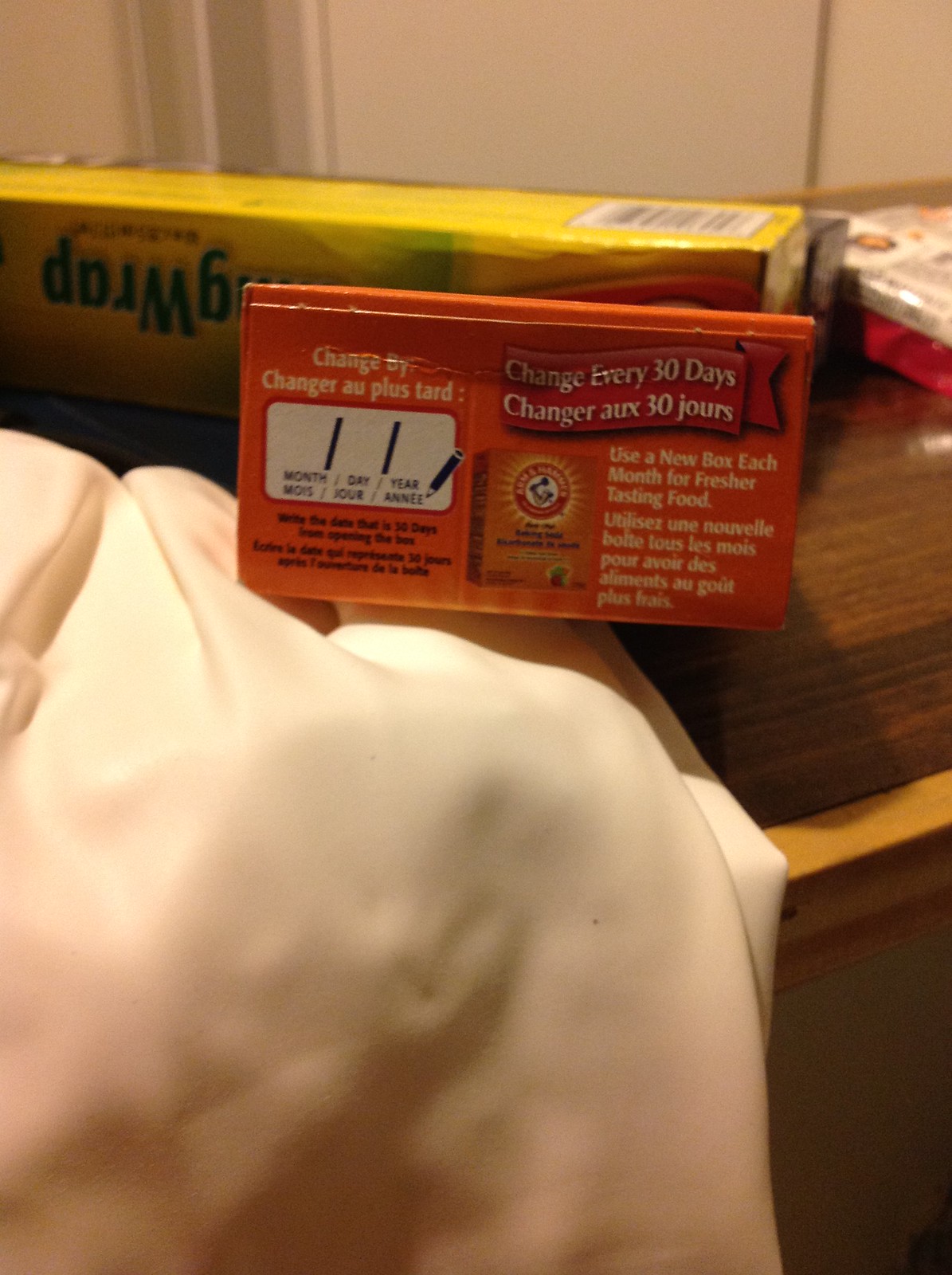This photograph captures a close-up of household items arranged on a dresser-like wooden surface. Dominating the foreground is a tipped-over box of Arm & Hammer baking soda, its familiar orange packaging clearly visible. The viewer's perspective shows the top of the box, which features a red banner with white text advising, "Change every 30 days," and the same instructions in French, "Changez aux 30 jours." Below, two white fields for month, day, and year are shown but remain blank. These instructional details are mirrored in both English and French. The baking soda box rests on a white cloth that is draped over the edge of the wooden surface, suggesting a casual setting.

In the background, an upside-down box of cling wrap with a distinctive yellow design is partially visible, hinting at additional household chores or organization. The blurred background also reveals vague shapes suggestive of more items or perhaps books, adding to the lived-in feel of the scene. The white wall behind these objects provides a neutral backdrop that contrasts with the colorful packaging of the household products.